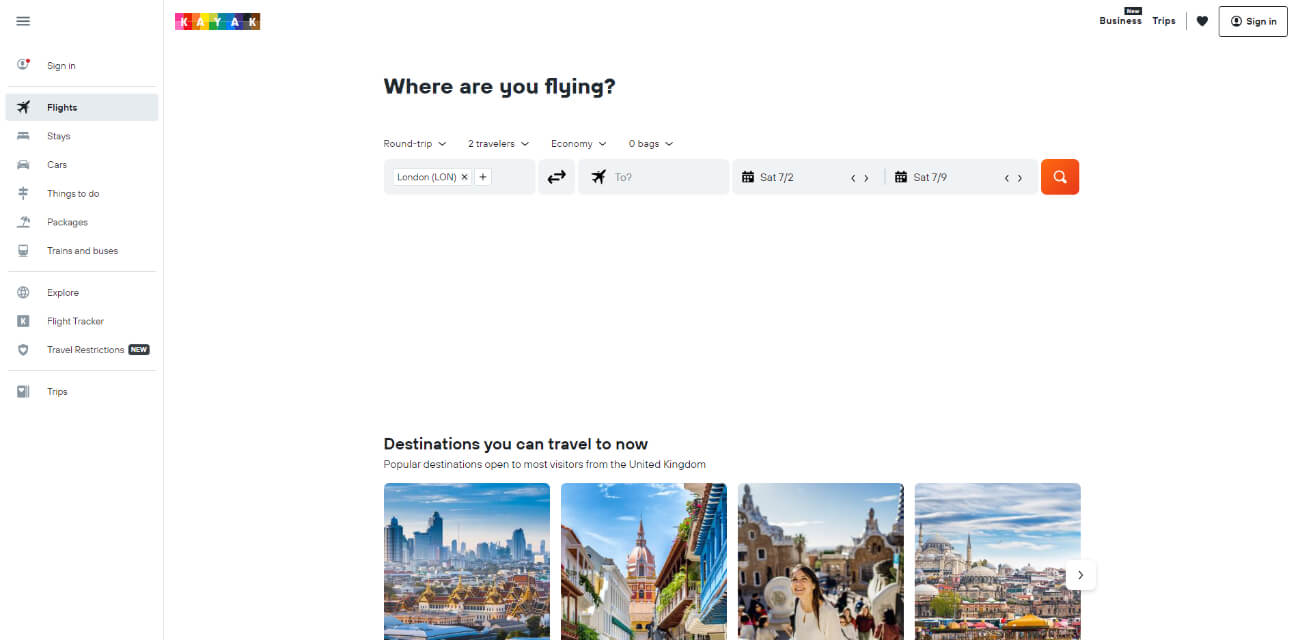This is a detailed screenshot of the website Kayak, a platform for booking travel itineraries, including hotels, flights, and rental cars. The user interface is divided into two main sections: 

- **Left Pane**: This column contains a vertical list of navigation options, each paired with a corresponding icon. The options include:
  - Sign In
  - Flights
  - Stays
  - Cars
  - Things to Do
  - Packages
  - Trains and Buses
  - Explore
  - Flight Tracker
  - Travel Restrictions
  - Trips

- **Right Pane**: This section, occupying the majority of the webpage, allows users to plan their trips. The prominent title "Where are you flying?" invites users to customize their travel plans. Key features include:
  - A row to adjust travel options, such as round trip, number of passengers, travel class (e.g., economy), number of bags, departure airport, destination, and travel dates.
  - A red 'Search' button for initiating the search.

At the bottom of the webpage, there is a row of four photographs under the heading "Destinations you can travel to now," showcasing popular destinations currently open to most visitors from the United Kingdom. Among the destinations, the last photograph appears to be from Turkey, with the others representing various global landmarks.